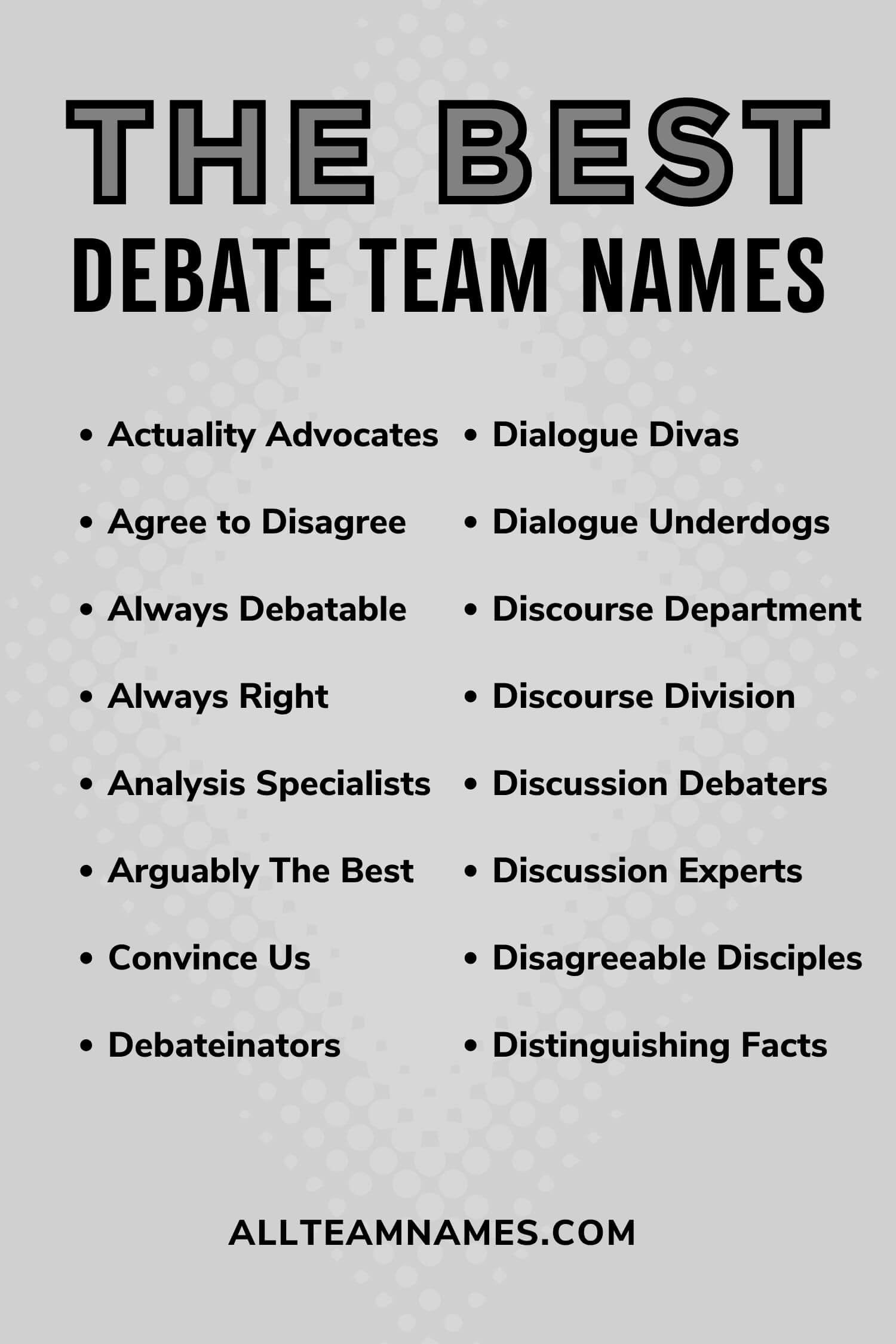The image features a poster with a light gray background adorned with a pattern of slightly darker gray circles, arranged in a subtle, diamond-shaped formation. At the top, in dark gray text with a black outline, the bold title reads "The Best Debate Team Names." Below the title, in simple black block letters, is a list of creatively named debate teams, including Actuality Advocates, Dialogue Divas, Agree to Disagree, Dialogue Underdogs, Always Debatable, Discourse Department, Always Right, Discourse Division, Analyst Specialist, Discussion Debaters, Arguably the Best, Discussion Experts, Convince Us, Disagreeable Disciples, The Debatenators, and Distinguishing Facts. Each name is accompanied by a corresponding black circle. At the very bottom, the source of the list is cited in black text as "allteamnames.com."